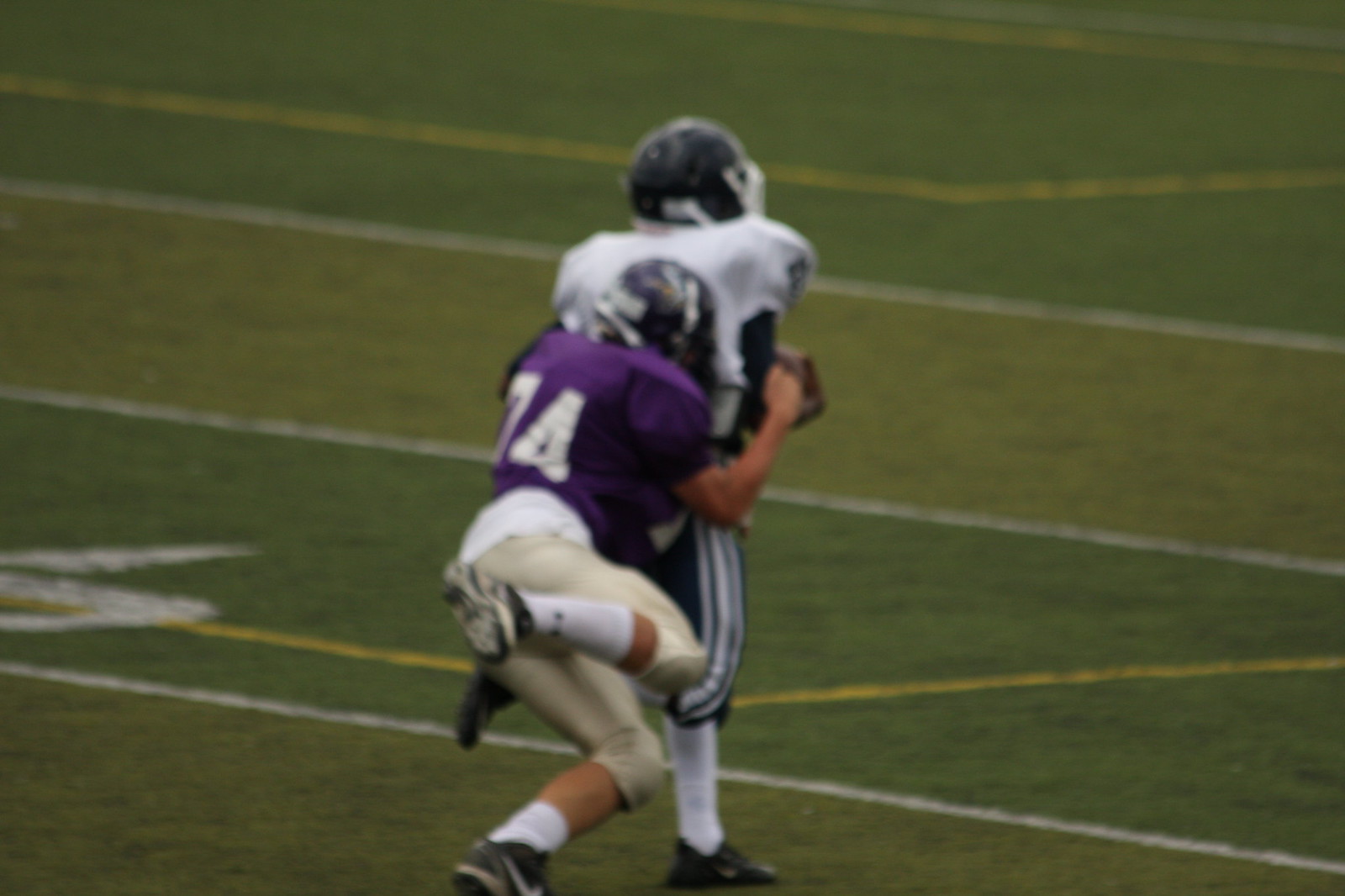The image is a color photograph taken outdoors on a green football field with white yardage stripes. The photograph captures a mid-play moment between two football players during a game. The player in the purple jersey, numbered 74, is mid-tackle behind the player in the white jersey and black pants with white stripes. The player in purple has white pants, black cleats, long white socks, and a black helmet. His right leg is in the air, indicating the dynamic action of the tackle, and his arms are wrapped around the player in the white jersey, pressing his helmet into the back of the tackled player. The photographed scene is closely focused on the players, emphasizing their intense physical struggle on the field. The tackled player appears to be holding a football in front of him, though only a small part of it is visible. The overall atmosphere suggests a decisive moment in the game.